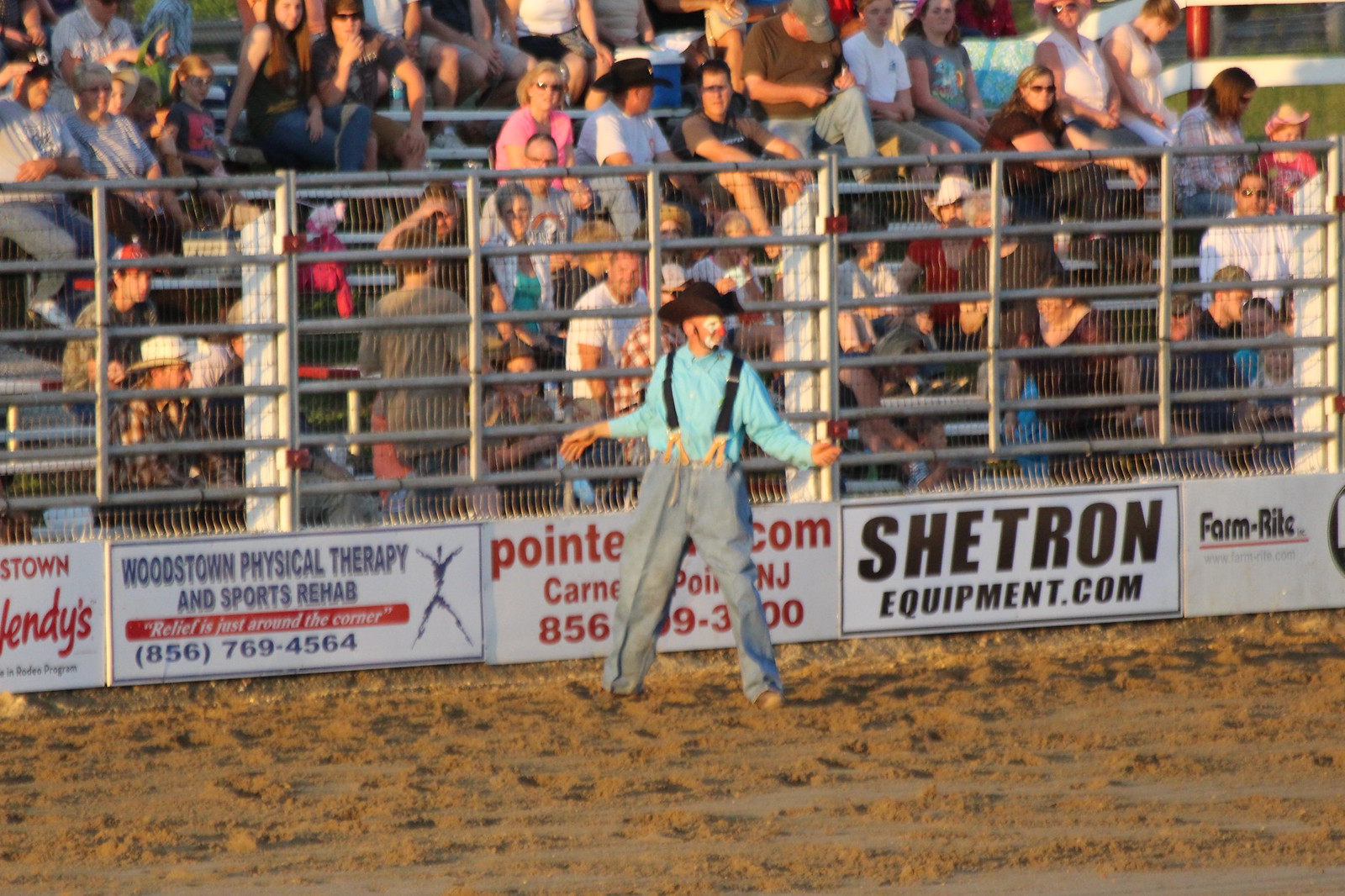In the picture, a rodeo event unfolds in a dirt arena. At the forefront, a rodeo clown is prominently featured. He is a Caucasian man wearing baggy blue jeans and black suspenders over a light blue, long-sleeved, button-down shirt. His head is topped with a black cowboy hat, and his face is adorned with clown makeup. He stands with his legs apart and arms outstretched, leaning slightly against a stockyard fence. Behind him stretches a large metal retaining wall, and beyond this wall, bleachers packed with spectators can be seen. The crowd, mostly seated, features some individuals wearing sunglasses and various colored hats. Along the bottom of the fence are several banners. The first banner is partially obscured but hints at being from Wendy's. The next reads "Woodston Physical Therapy and Sports Rehab," followed by "Relief is just around the corner," alongside a figure drawing and the phone number 856-769-4564. Another banner beside the clown is unreadable due to his position. To the right, two more banners are visible: "SheepRunEquipment.com" and a partially cut-off "Farm Right". The atmosphere is bustling, capturing the vibrancy and excitement of the rodeo event.